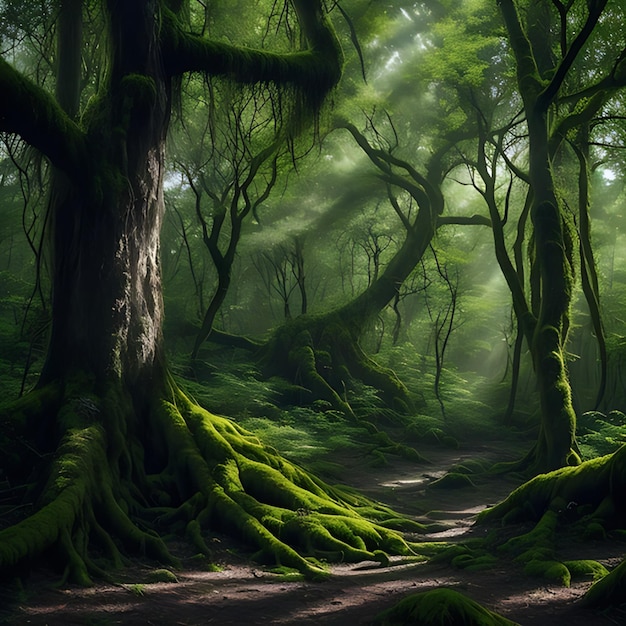This digital fantasy artwork showcases an eerie, green-hued forest scene enveloped in a vibrant, almost surreal greenness, reminiscent of a fantasy movie setting. Dominating the left side of the image is a large tree with a thick trunk and roots covered in green algae or grass. Scattered throughout the scene are other similar trees, most of which also have algae creeping up their trunks and branches. A sandy, brown path meanders from the foreground and disappears into the distant depths of the forest, enhancing the mysterious atmosphere. Sunlight barely filters through the dense canopy above, illuminating patches of leaves and casting a soft, ethereal glow on the forest floor. This intricately detailed artwork creates an enchanting, otherworldly environment that feels both inviting and enigmatic.